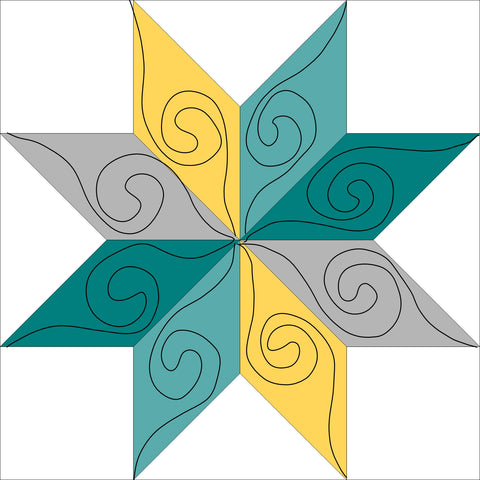The image features a meticulously designed pinwheel-shaped star with eight evenly spaced points, displayed against a white background. Each point reflects one of four repeating colors: light purple, dark green, lighter aqua green, and gold. The symmetrical design ensures that each pair of opposing points shares the same color. A subtle black line borders the entire image, enhancing its geometric precision. Each colored section within the star contains a distinct black swirl that loops from the center, adding an intricate touch to the overall graphic. This digital artwork, characterized by its balanced composition and vivid hues, exhibits a perfect blend of symmetry and elegance.